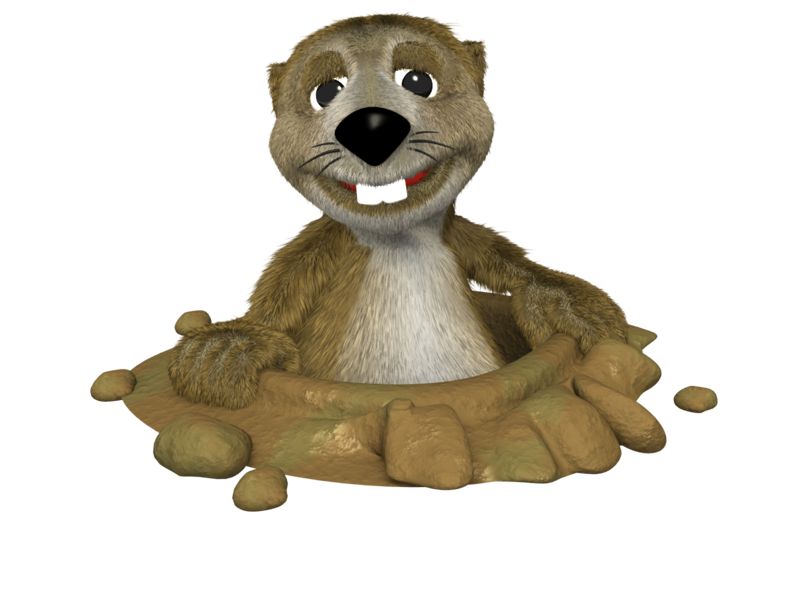The image presents an adorably animated, AI-generated cartoon gopher, emerging from a muddy, dirt-brown hole set against a pristine white background. The gopher, bearing a close resemblance to a prairie dog, showcases a fur coat with light brown hues interspersed with darker brown shades and a whitish-tan belly. Its face exudes a sense of friendly, albeit slightly melancholic charm with droopy black eyes, a prominent and very black nose accentuated by three whiskers on each side, and a wide, somewhat fake smile. This smile prominently features two large, sparkling white buck teeth and a glimpse of its red tongue. Its cute, small hands enhance its soft and inviting appearance, ideal for a children's cartoon. Scattered around the hole are small, pebble-like bumps and slight hints of olive green, enriching the dirt's natural texture. The background’s stark white simplicity ensures the gopher remains the focal point, emphasizing its endearing expression and overall cartoonish appeal.